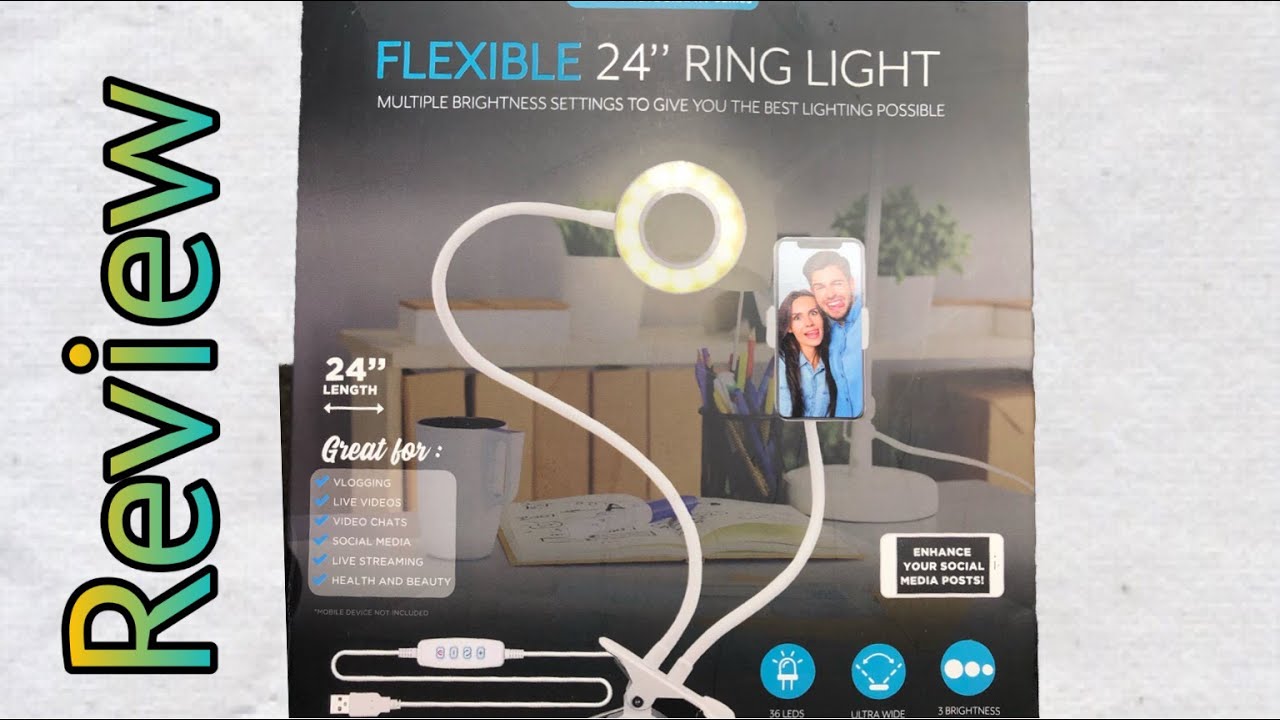The image features a grey background with the word "REVIEW" prominently displayed on the left side in a vertical orientation, starting with "R" at the bottom and ending with "W" at the top. The text gradient transitions from yellow to green to blue as it progresses from bottom to top. 

Central to the image is a detailed advertisement for a "FLEXIBLE 24-inch ring light." The ring light is characterized by its multiple adjustable brightness settings designed to provide optimal lighting. The device is shown radiating a bright white light and is equipped with flexible, bendable arms, ending in a circular light source. One of its arms is holding a smartphone displaying a photo of a man and a woman.

Text within the image highlights its features and uses, including "24-inch lamp," "great for live video, video chat, social media, live streaming, health and beauty," and it encourages users to "ENHANCE YOUR SOCIAL MEDIA POST." The product also comes with a cable and includes three blue circles containing additional information.

Overall, the caption gives a comprehensive overview of the ring light's functionality and benefits, emphasizing its versatility and suitability for various digital content creation activities.